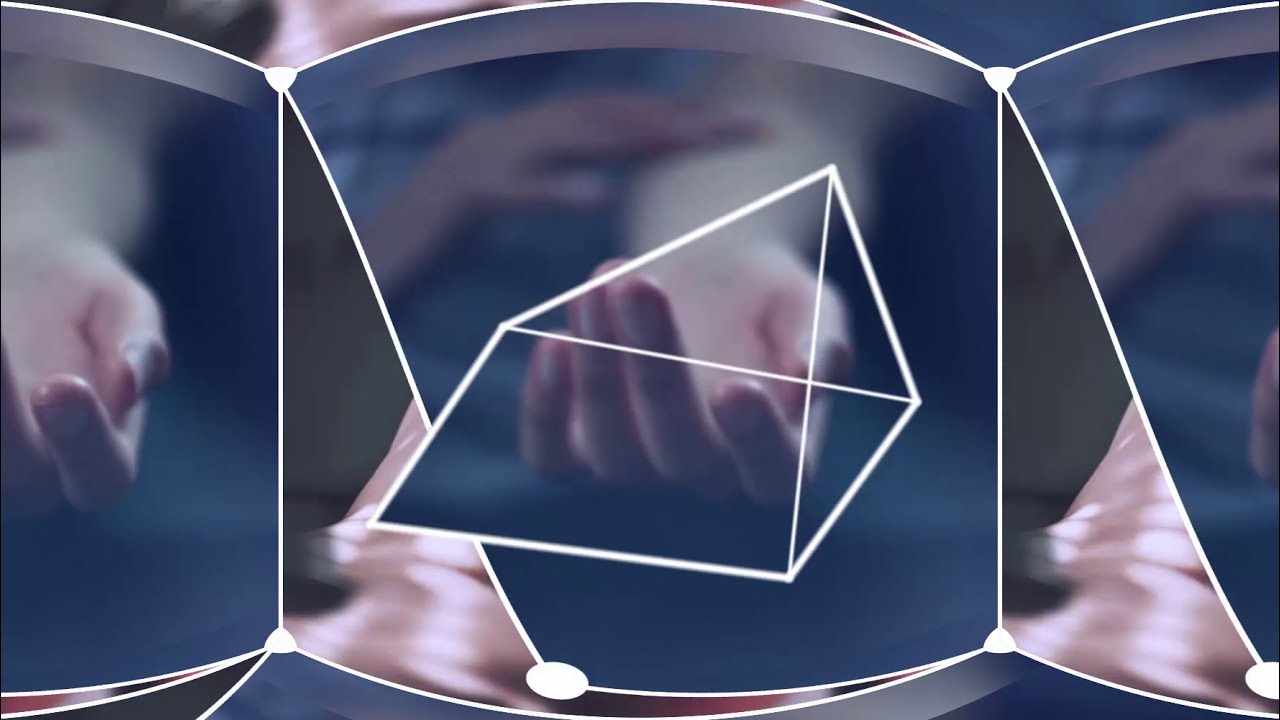This detailed and enigmatic image captures an array of human hands intertwined and positioned in various ways within a complex geometric design. The central focus is a realistically depicted hand with its palm facing up and fingers gently curled, suggesting a tender posture. Surrounding this central hand are additional hands, some holding each other, contributing to a sense of unity or connection. The scene is enveloped in a plethora of geometric shapes, such as triangles, hexagons, and rectangular prisms with curved edges, creating a layered and intricate backdrop. White lines delineate these shapes, segmenting the image into fragmented yet interconnected parts. A blue background subtly contrasts with the warm tones of the hands, adding depth and visual interest. The composition is complemented by areas of distortion, where the hands and fingers appear duplicated or partially visible, almost as if they are emerging from or blending into the geometric forms. Among these elements, there are hints of plaid fabric, possibly suggesting the presence of a person just behind or intertwined with the hands. This artistic piece, awash with symbolic complexity, merges human touch with abstract geometry, offering a thought-provoking visual experience.